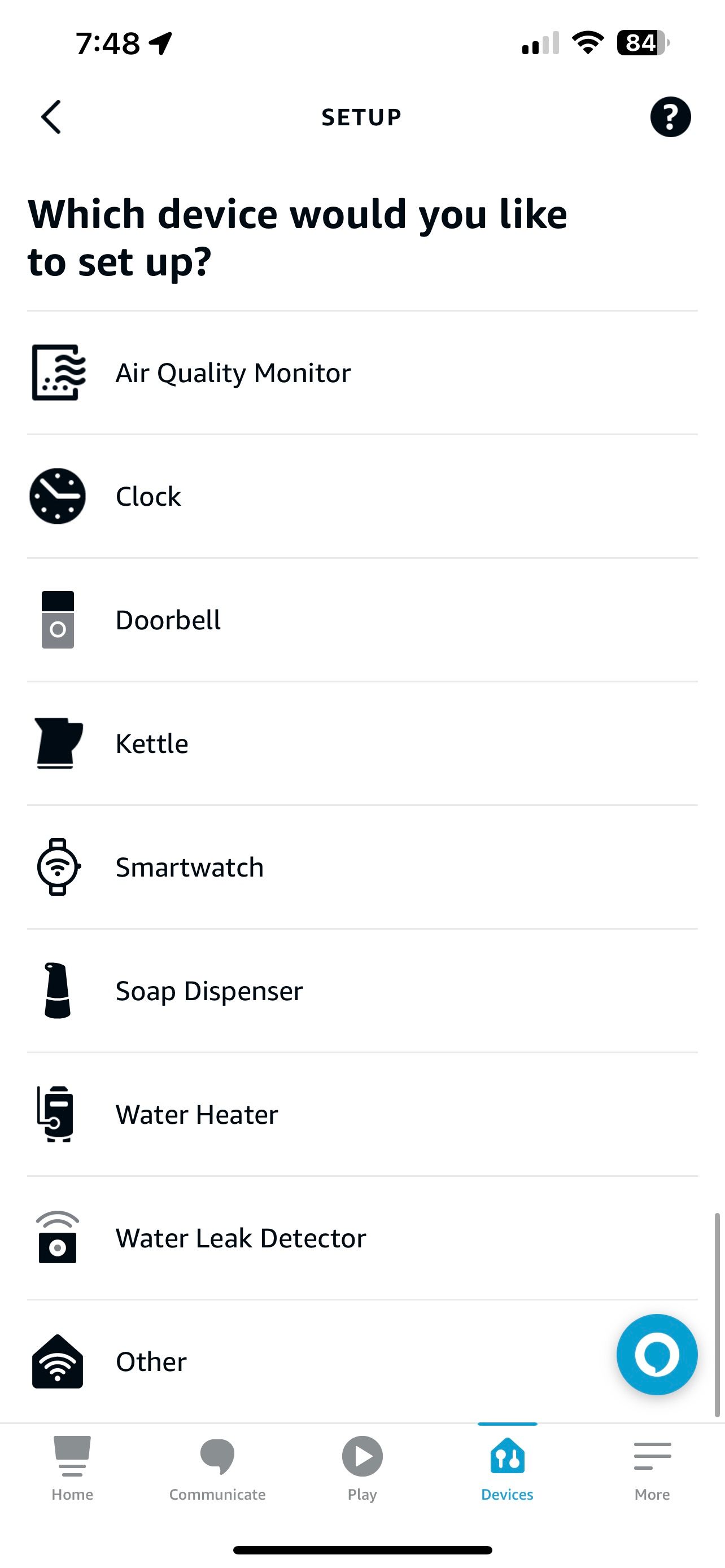The screenshot displays the interface of a smartphone. In the top left corner, the time is shown as 7:48, accompanied by a location icon. On the top right side, there are icons indicating cell signal strength, Wi-Fi connection, and a battery level at 84%. Below this, there is a horizontal bar with a left-facing arrow < symbol on the left, the word "Setup" centered, and a question mark icon on the far right.

The main section of the screen is titled “Which device would you like to set up?” followed by a list of device options, each preceded by an icon. The options include: 

1. Air Quality Monitor
2. Clock
3. Doorbell
4. Kettle
5. Smartwatch
6. Soap Dispenser
7. Water Heater
8. Water Leak Detector
9. Other

Navigational buttons are located at the bottom of the screen. From left to right, these buttons are: Home, Communicate, Play, and Devices (represented by a blue house icon). Additionally, a "More" menu is available, above which is the Amazon Alexa icon.